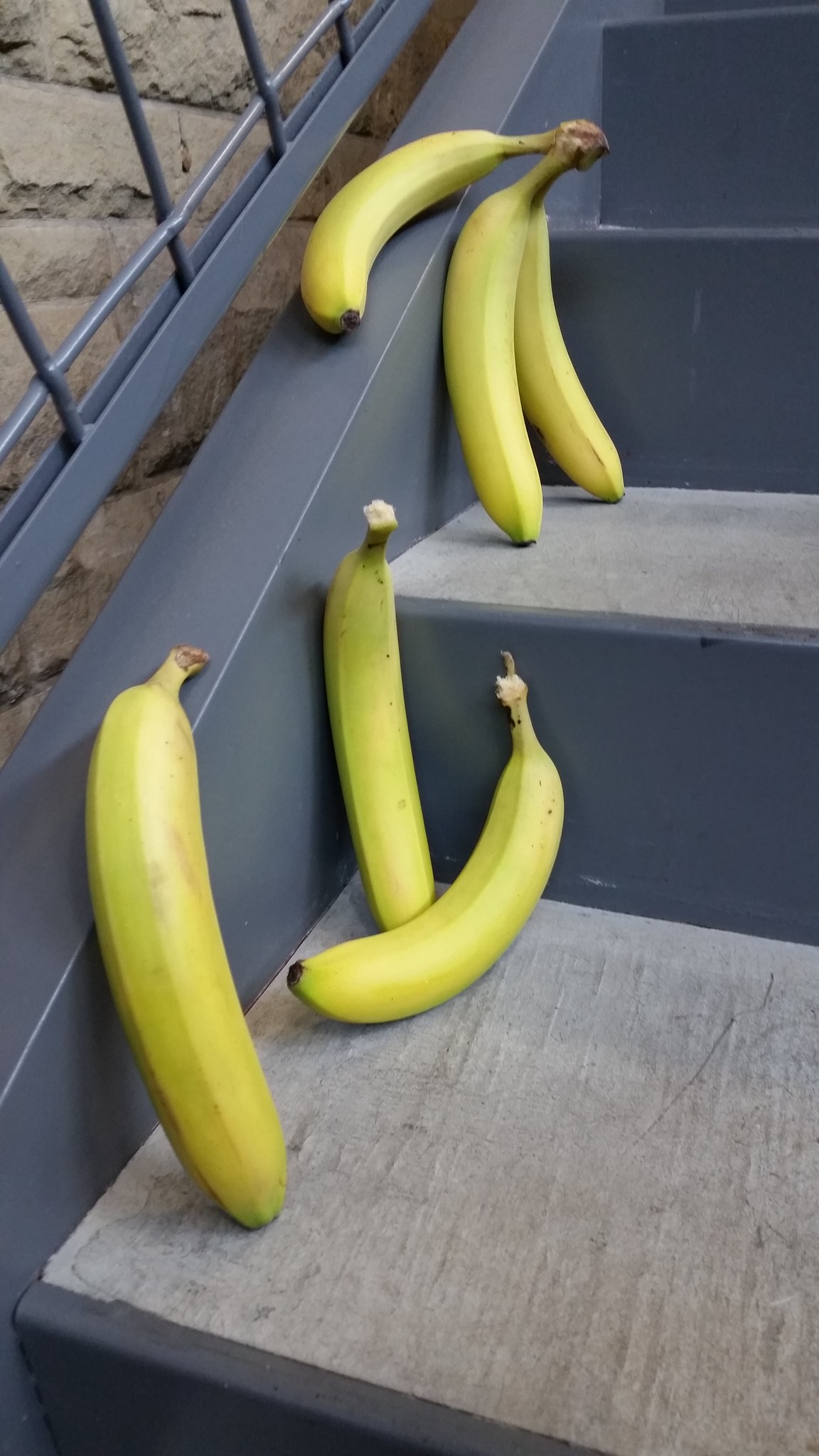The photograph features a stairwell scene with a collection of bananas at different stages of ripeness, mainly yellow with a hint of green. The staircase comprises gray concrete steps, framed by a gray metal railing on one side, and a rough-hewn brown brick wall with gray mortar on the other. The lower section of the scene shows three loose bananas positioned on the bottom step: one lying on its back with its curve up, another standing with the back of its curve facing us, and the third propped in the corner with its front curve visible. Moving up the stairs, the next step holds a bunch of three bananas still connected at the stem, leaning against the side rail with their inside curves facing right. This detailed image, appearing well-lit possibly due to natural light, allows for a close-up view of the bananas arranged on the steps, highlighting their slightly underripe condition without any spots or blemishes.